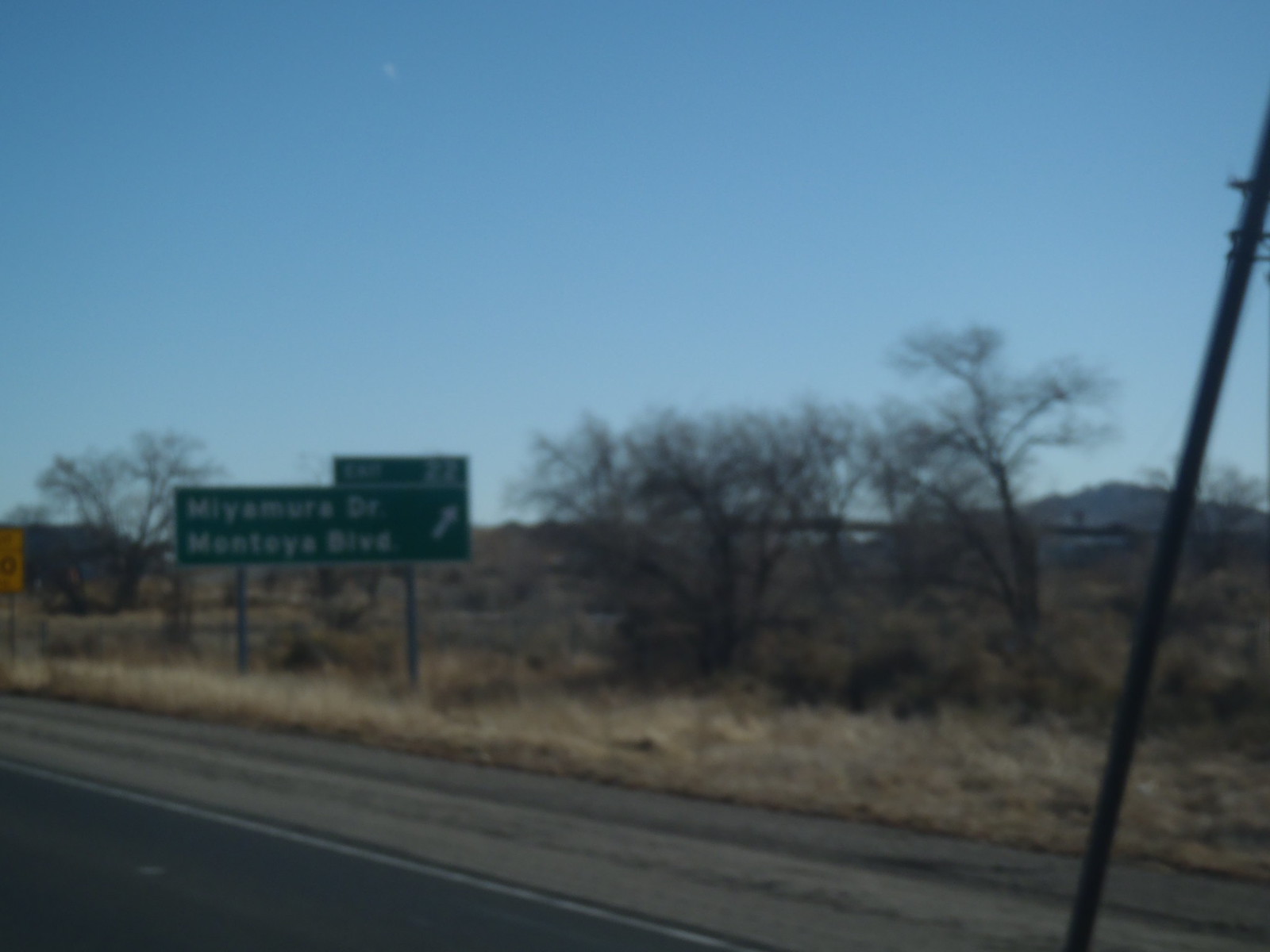The image captures a countryside scene from a moving car on a highway. The picture is slightly blurry, indicating either the camera was in motion or an older model was used. Along the dark gray road, the shoulder is lined with dead brown grass and barren, craggy trees. Dominating the scene is a green highway sign with white text, mounted on steel supports. Despite the blurriness, the sign seems to say "Miamra Drive" and "Montoya Boulevard," with an arrow pointing to the right and indicating Exit 22. Above, the sky is a strikingly clear and vibrant blue, devoid of any clouds. The overall landscape lacks much detail, evoking a sense of isolation and open space.